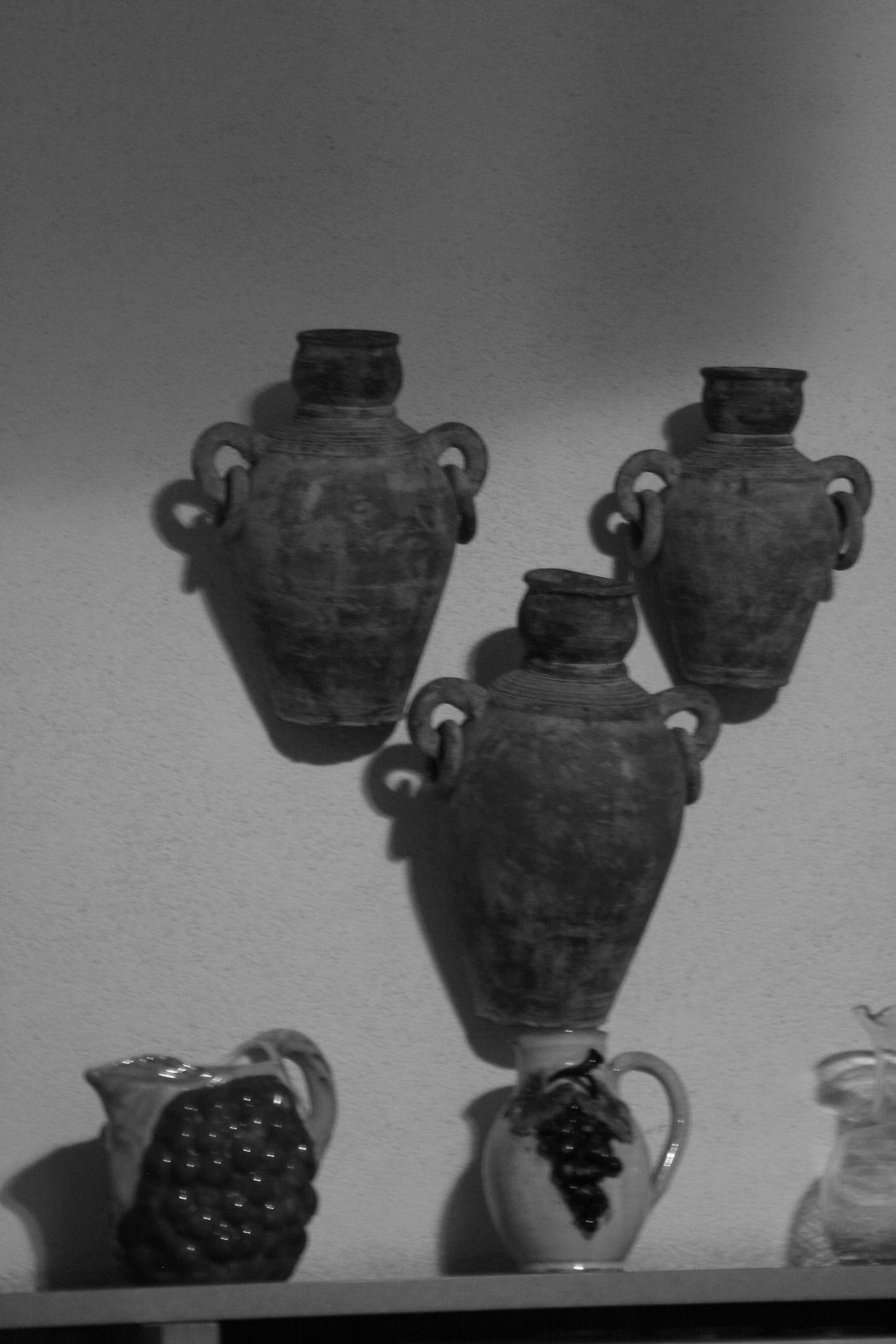This black and white photograph showcases a striking arrangement of ceramic teapots and urns against a light-colored wall. At the bottom of the image, three distinct ceramic teapots sit elegantly on a light-colored shelf, with their spouts oriented towards the left. Each teapot features a detailed, raised design resembling clusters of grapes and grape leaves. The leftmost teapot is shaped like a bunch of grapes with textured, bumpy bubbles and a handle that resembles grape leaves, while the middle teapot is adorned with a grape motif and metallic accents on its handle, base, and lip. The rightmost teapot, only partially visible, appears to be a clear glass pitcher.

Above the shelf, three urns, reminiscent of ancient amphorae, are mounted on the wall in a triangular configuration—two at the top and one at the center below. These urns, likely designed as plaques, exhibit the traditional urn shape with rounded U-shaped handles connected by circular interlocking rings. The urns, slightly varied in size, evoke a sense of antiquity and museum-like quality, adding to the overall historical and artistic ambiance of the image. The grayscale tones of the photograph enhance the textural contrasts and intricate details of the ceramics, making the scene appear both timeless and elegant.